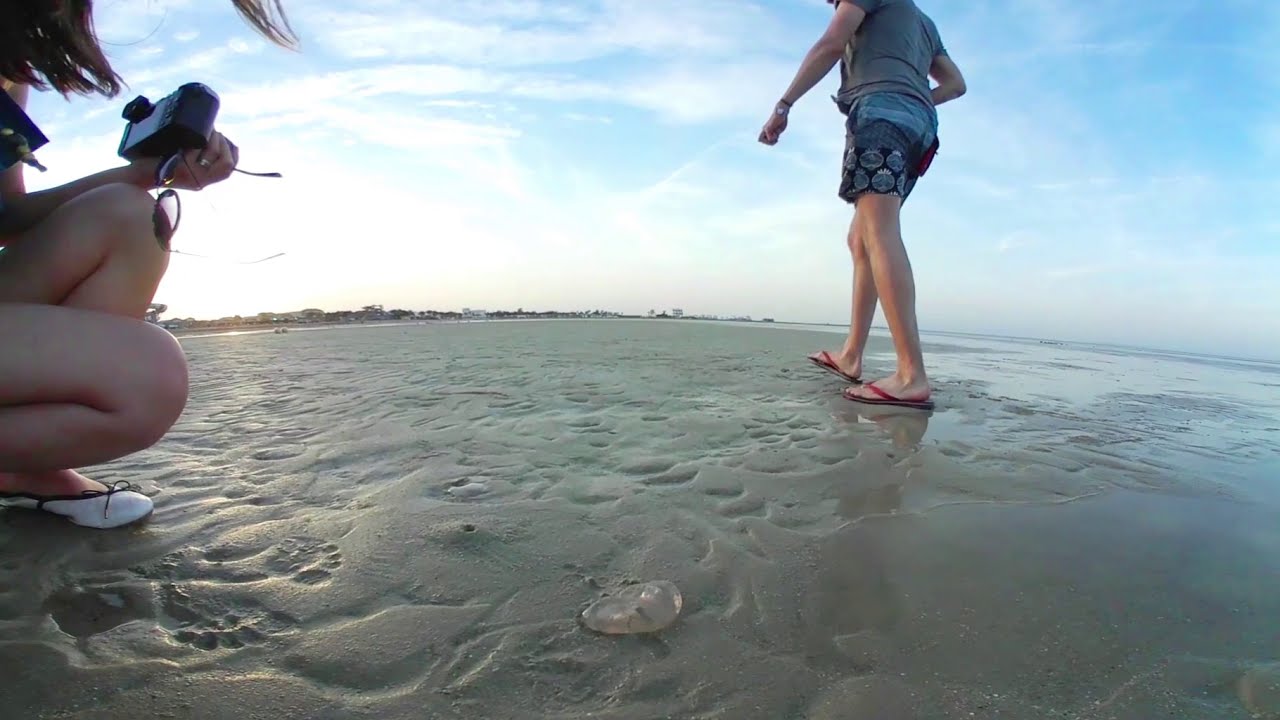The image captures a serene beach scene under a bright, partly cloudy blue sky. Two young girls are featured prominently. The girl on the right, seen from a low ground-level perspective, is walking in the shallow, wet sand left by the receding tide. She dons red sandals, blue shorts with a flower pattern, and a layered shirt consisting of a darker gray outer layer over a lighter blue one. Her right arm is bent toward her body, while her left arm swings out, adorned with a watch. Her right leg is raised mid-step, with her left leg firm on the ground. On the left side of the image, another girl with shoulder-length brown hair is kneeling, perhaps to take a picture with the large-lensed camera she holds in her left hand. She also clutches her glasses and is wearing white shoes. The sand is a light brown color, and there's a minor detail of a jellyfish or water sack nearby in the foreground. The horizon shows a distant tree line, adding to the tranquil coastal atmosphere.